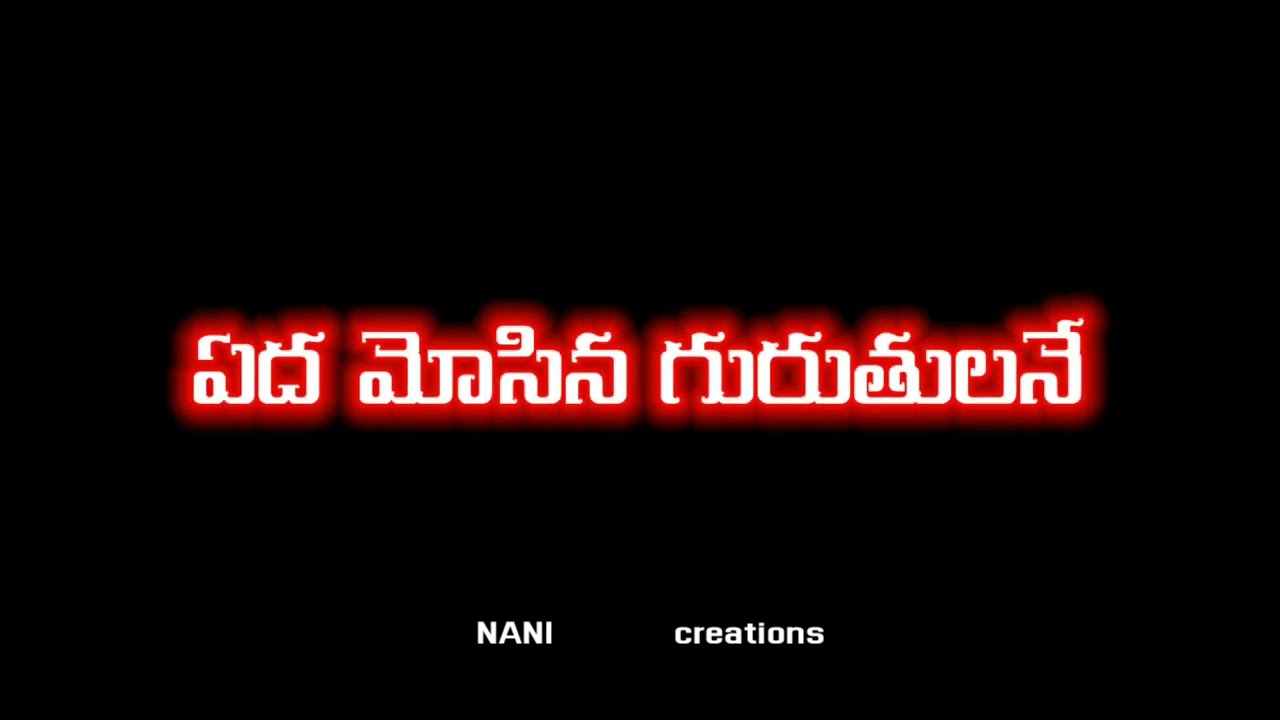The image features a rectangular black background with prominent text in the center and additional text at the bottom. The central text is in a foreign language, printed in white with light berry-red outlines that resemble a glowing effect. Each letter has a unique design with curved corners and some featuring a small pipe-like detail at the top. Below this, near the bottom middle of the image, the words "NANI" and "creations" are printed in white. "NANI" is in bold, all-uppercase letters, while "creations" is in lowercase letters, with a noticeable gap between the two words.